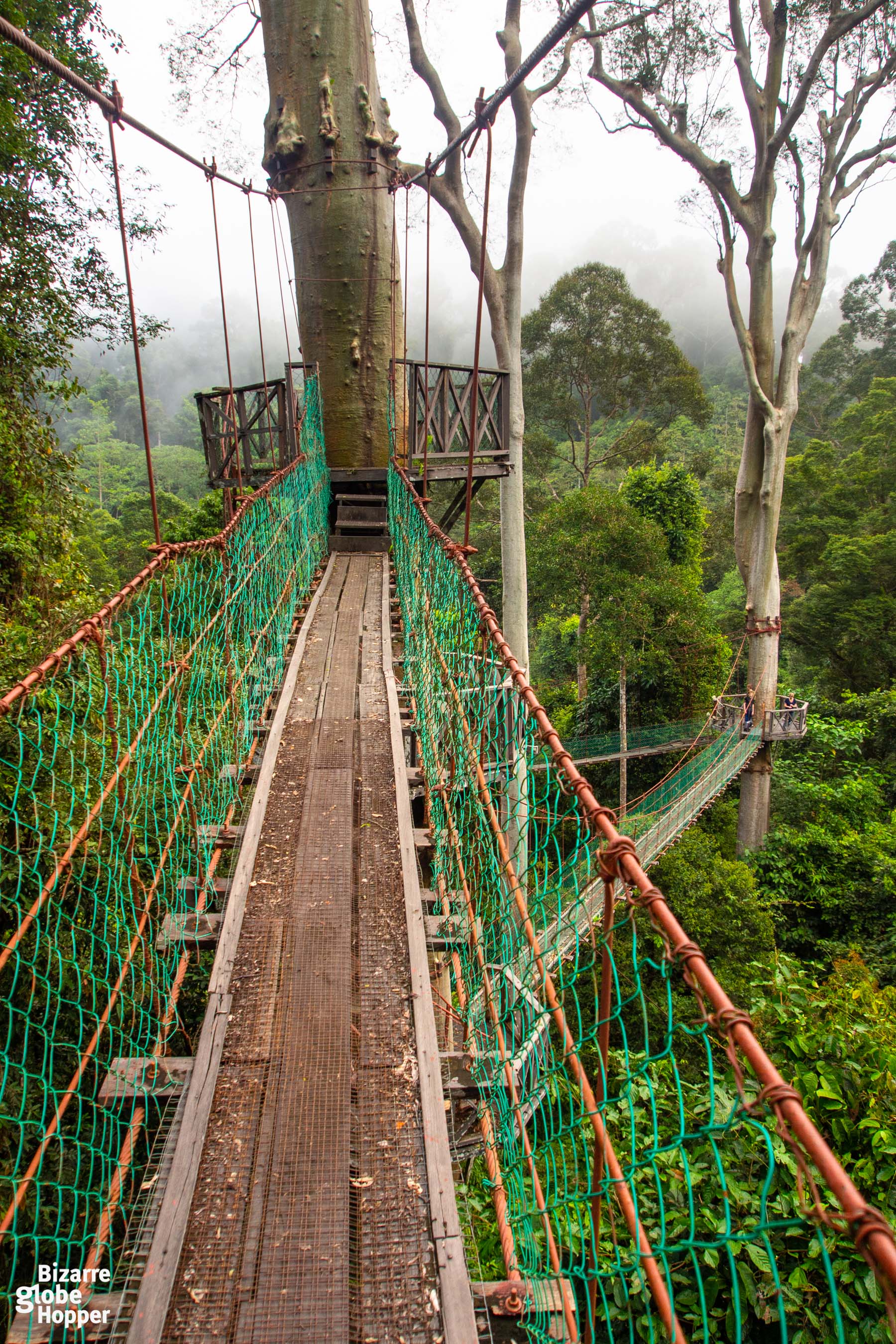The image depicts a suspended wood-planked walkway traversing a densely forested area, with the footbridge receding from the bottom center to the back center. The walkway, flanked by green netting for protection, leads to a set of stairs ascending to a wooden platform with intricate railings forming X-shaped cross posts. Dominating the center of this platform is the large trunk of a towering, brown tree. The scene, set amidst a fog-laden, heavily wooded environment with tall and mostly bare trees, shows elements of a tree climbing or ropes course. Additional platforms and course features are visible, including another prominent tree trunk on the right, underscoring the bridge's connection to multiple pathways. Below the elevated walkway, a dense canopy of green foliage stretches out, enveloped under a white sky.